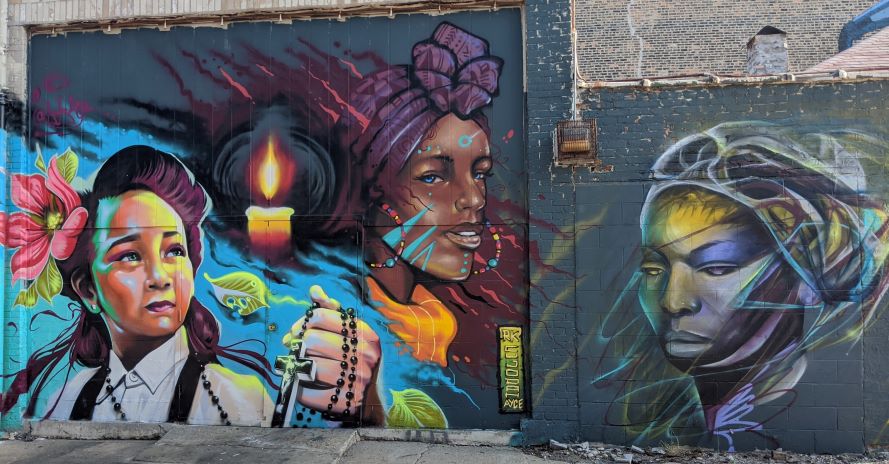The image showcases a highly detailed mural painted on a brick wall, seemingly commissioned given its artistic quality. On the left side of a large garage-style door, the mural features a striking depiction of a woman with a red flower in her hair. She is looking up and slightly to the right, wearing a white shirt with visible straps over her shoulders. Above and to the right of her head is a lit candle, contributing a symbolic depth to the artwork. Surrounding her are leaves and a background accented in blue hues, with a hand holding a rosary featuring a cross to her right.

The central part of the mural, positioned on the door, portrays another woman with a purple bow in her shorter hair. She is facing right, adorned in a yellow shirt that appears turtleneck-like, with purple elements framing her face. Her image is set against a backdrop transitioning to dark gray. At the bottom right of the door, there is some illegible writing.

To the right of this door, on the lower half of the wall, another woman's visage is painted, looking slightly down and to the left. The simplicity of her portrayal, defined by black and white lines with blue accents around her face and purple lines below her neck, creates a somewhat enigmatic presence. Above her, a small, box-like object is affixed to the gray brick wall, possibly a power box. The mural's upper portion displays white netting stretched across the wall, disappearing off the image frame on both the top and right sides.

The mural, while vibrant and intricate, appears against a dark teal or dark blue background, suggesting a contrast that highlights the detailed artwork. The artist, likely possessing considerable talent, may focus on depicting individuals with distinct features, possibly indicative of African descent, given the characteristics observed. The overall setting includes a glimpse of gray concrete pavement at the bottom of the image, tapering off towards the right.